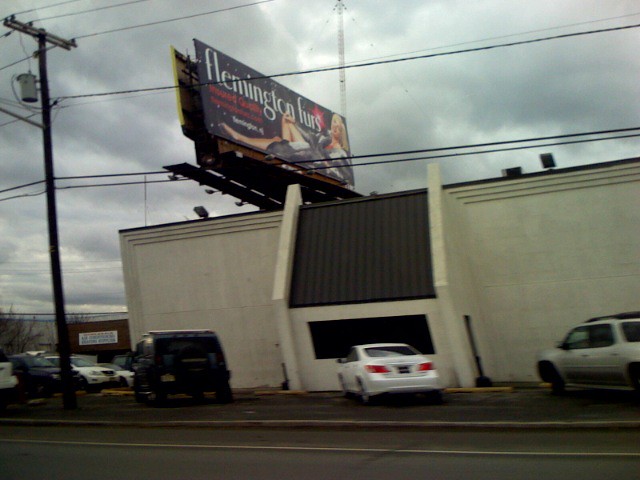In this slightly blurry outdoor image, a gloomy atmosphere is created by the very dark clouds overhead, suggesting an impending rainstorm. The scene features a stucco-covered building with a prominent large window on its visible side. No doors are in sight, indicating they are likely situated on the opposite side of the structure. Adjacent to this building are designated parking spaces, reinforcing the idea that it is situated within a larger plaza, as other buildings are also visible in the background. A few cars are parked around the corner, adding to the urban setting. A telephone pole stands nearby, and perched atop the building is an enormous billboard. The billboard dominates the scene with its size relative to the building and depicts a woman reclining in a fur coat. Red lettering is also present on the billboard, but the angle of the image prevents it from being legible.